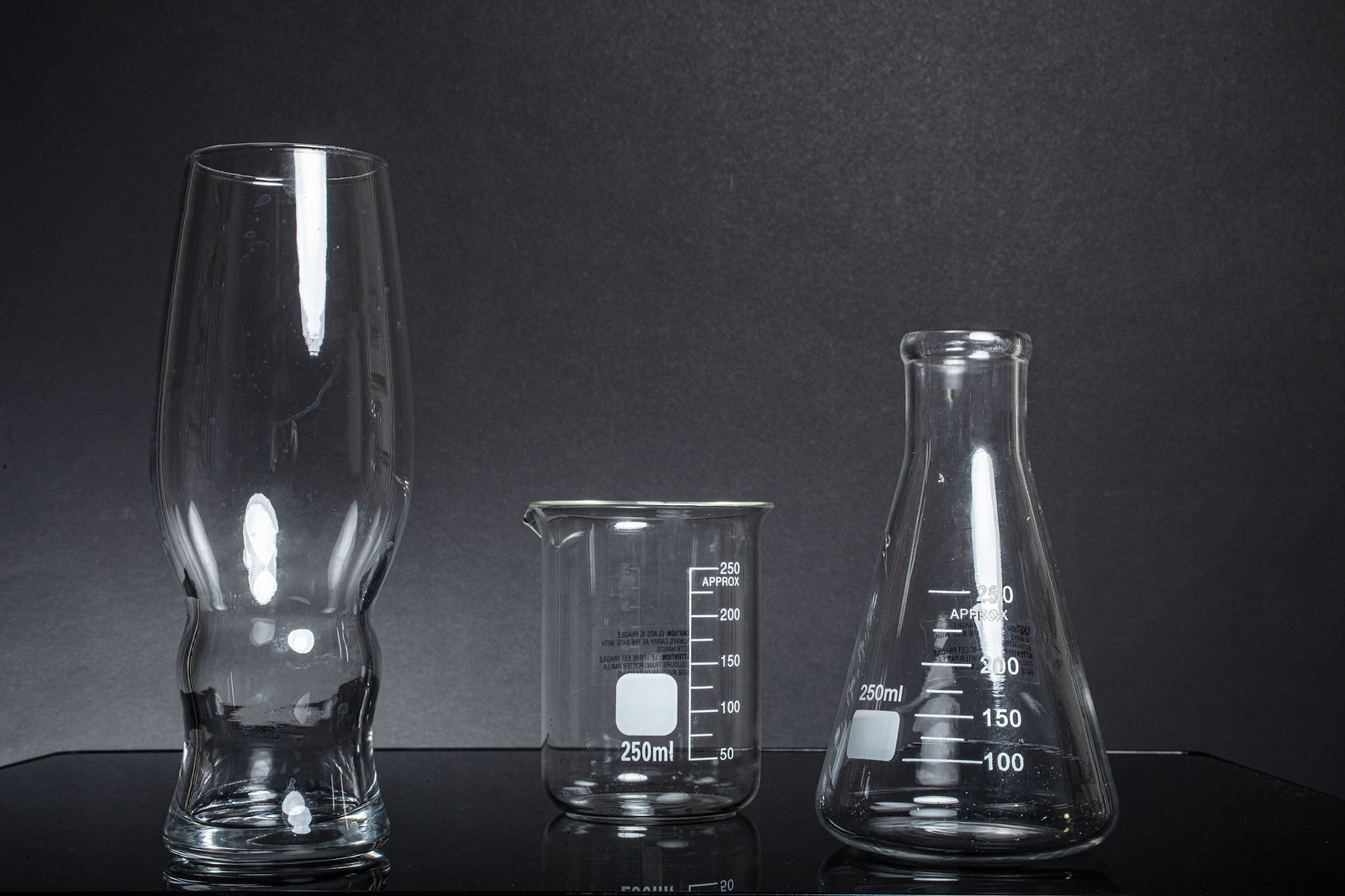This black-and-white photograph features three distinct pieces of glassware set against a dark surface with a plain, dark gray wall in the background. On the left is an intriguing glass resembling a pint glass, with a wide base that narrows slightly before flaring out at the top. While it appears suitable for quick measurements or even as a beverage glass, it lacks any numerical gradations. The middle item is a typical wide-mouth beaker marked for 250 milliliters, with graduation lines descending from 250 down to 50 milliliters. On the right is an Erlenmeyer flask, also marked for 250 milliliters, with graduation lines from 250 down to 100 milliliters. The reflective surfaces of all three glass objects catch the light and add a touch of elegance to the otherwise utilitarian laboratory equipment.